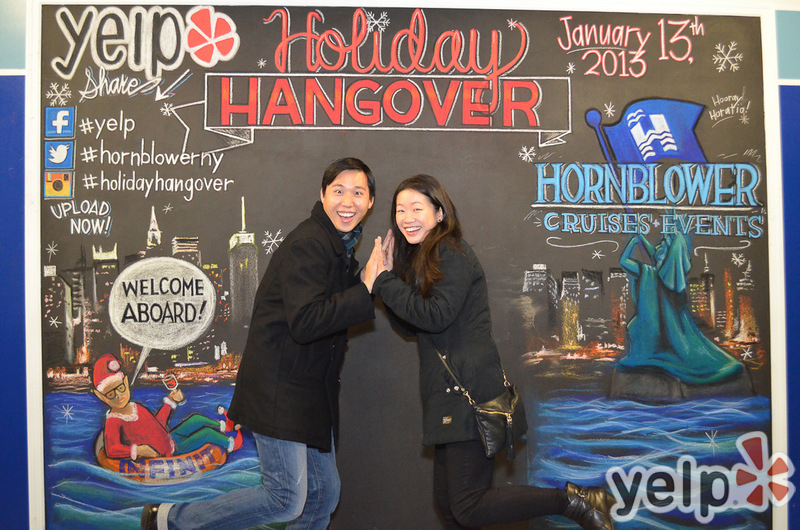The photograph features a young Asian couple, a man on the left and a woman on the right, centered against a large chalkboard backdrop. Both are standing on one foot with hands clasped together and smiling, creating a playful pose. They're dressed in black winter jackets, and the woman carries a black purse over her shoulder. Above them, written in red and white script, are the words "Holiday Hangover" with a white snowflake dotting the 'i' in "Holiday." The event date, "January 13, 2013," is chalked in white with a red outline on the right side of the image. 

To the far right, a greenish-teal caricature of the Statue of Liberty holding a flag with a blue banner and a white 'H' logo can be seen, and further up, snowflakes are chalked into the backdrop. In the bottom left corner, an elf dressed as Santa is floating in an orange inner tube, holding a wine glass and a speech bubble saying "Welcome aboard." The lower right corner prominently displays the Yelp logo in black lowercase script outlined in white. Additional logos for Facebook, Twitter, and Instagram are positioned in the left corner, represented by their respective icons: a blue square with a white 'F' for Facebook, a blue square with a white bird for Twitter, and a camera icon for Instagram.